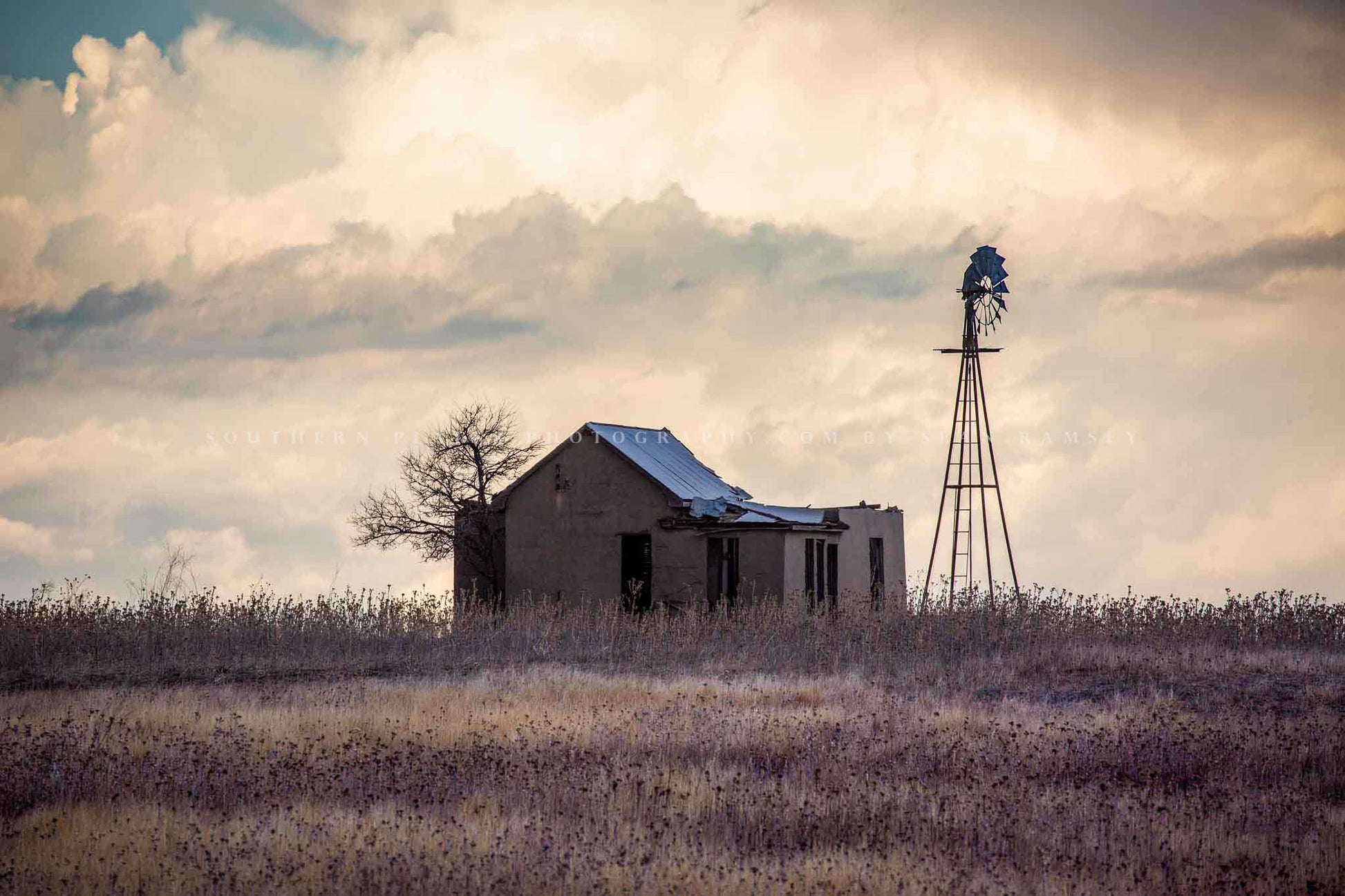The photograph captures an outdoor scene of an old, dilapidated stone shed situated on farmland. The roof of the shed appears to be partially collapsed, and its weathered blue shingles are visible. To the left of the shed stands a barren, leafless tree, while to the right, a tall structure with a ladder supports a small windmill, typical of those found on farms. The foreground is dense with very tall, thin grasses of varying shades, from light tan to yellow, interspersed with clusters of reddish flowers, creating a tapestry of colors in the bottom third of the image. The sky above is dominated by an expansive mass of clouds tinged with faint hints of orange and gray, with a few patches of bright blue visible in the upper left corner. The horizon is sharply defined by the massive cloud, which fills up the upper portion of the photograph. A faint, blurry watermark that reads something like "something photography" can be made out in the center of the image.